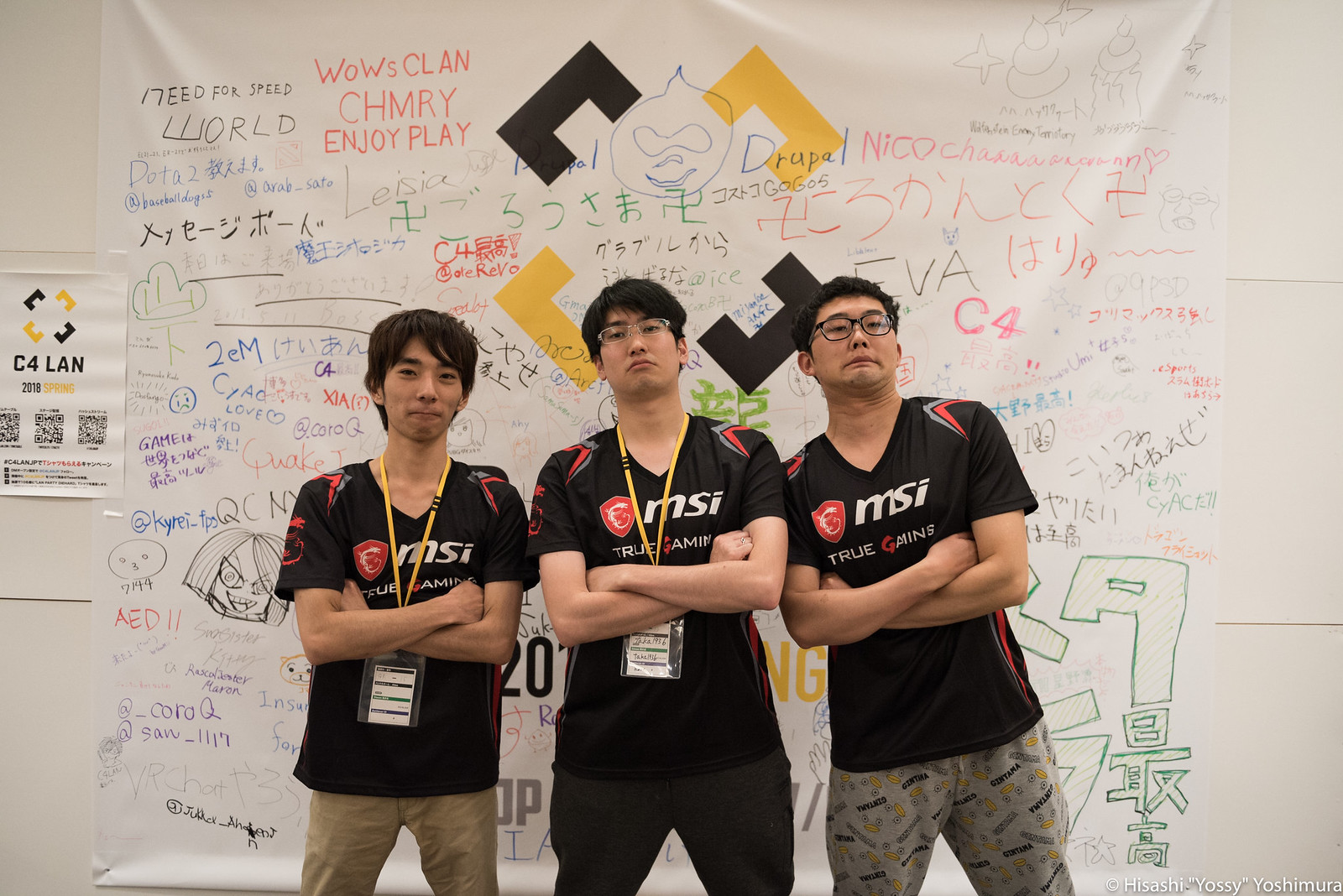Three Asian men pose in front of a large white sheet covered with a plethora of handwritten messages and doodles, some in English, such as "Need for Speed," "WoW's Clan Chivalry," and "Enjoy Play," and others likely in various Asian languages. The men stand with their arms crossed, exuding a sense of camaraderie and playfulness, especially the ones on the ends. Two of them are wearing glasses. They all sport matching black jerseys branded with the MSI logo, a red shield, and the words "True Gaming" in red. The man on the left stands next to a smaller sheet of paper that also features the MSI logo beside the text "C4 LAN 2018." Below the MSI logo on this sheet, there are additional smaller texts and QR codes that are difficult to decipher. The central white sheet suggests a community vibe, likely linked to a gaming event or LAN party, giving off a spirited and enthusiastic atmosphere.